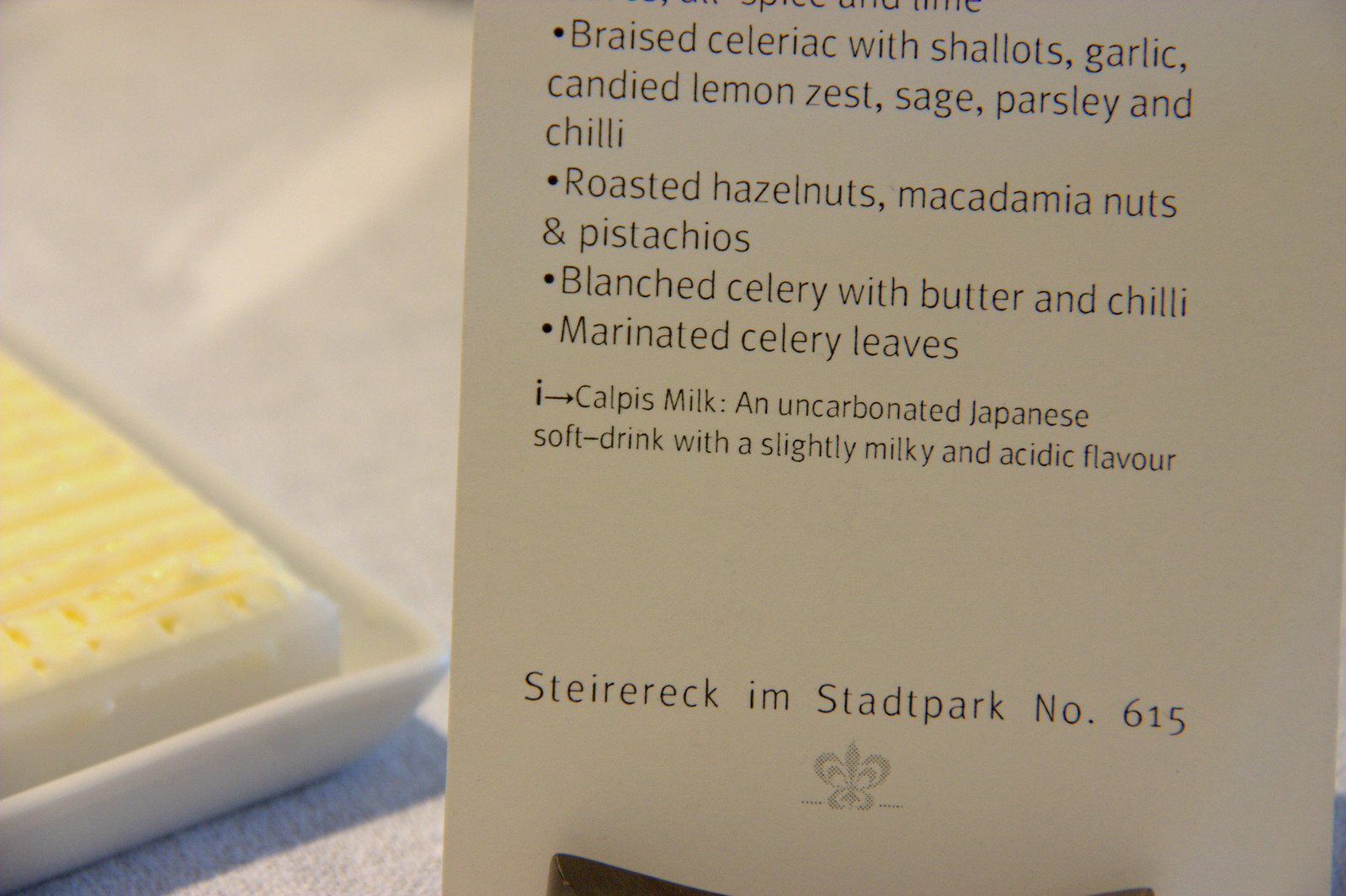The photograph features a partially visible buffet menu card standing upright, held in place by a wooden holder at the bottom. To the left of the menu card, there is a white dish containing what appears to be food, possibly cheese or cake, positioned on a white tablecloth. The text on the menu card includes the following detailed items: braised celeriac with shallots, garlic, candied lemon zest, sage, parsley, and chili; roasted hazelnuts, macadamia nuts, and pistachios; blanched celery with butter and chili; marinated celery leaves. Additionally, there is an explanation of Calpis milk, described as an uncarbonated Japanese soft drink with a slightly milky and acidic flavor. At the bottom of the menu card, it notes "Steric M. That's park number 615," accompanied by artwork resembling a crown rendered in dots.